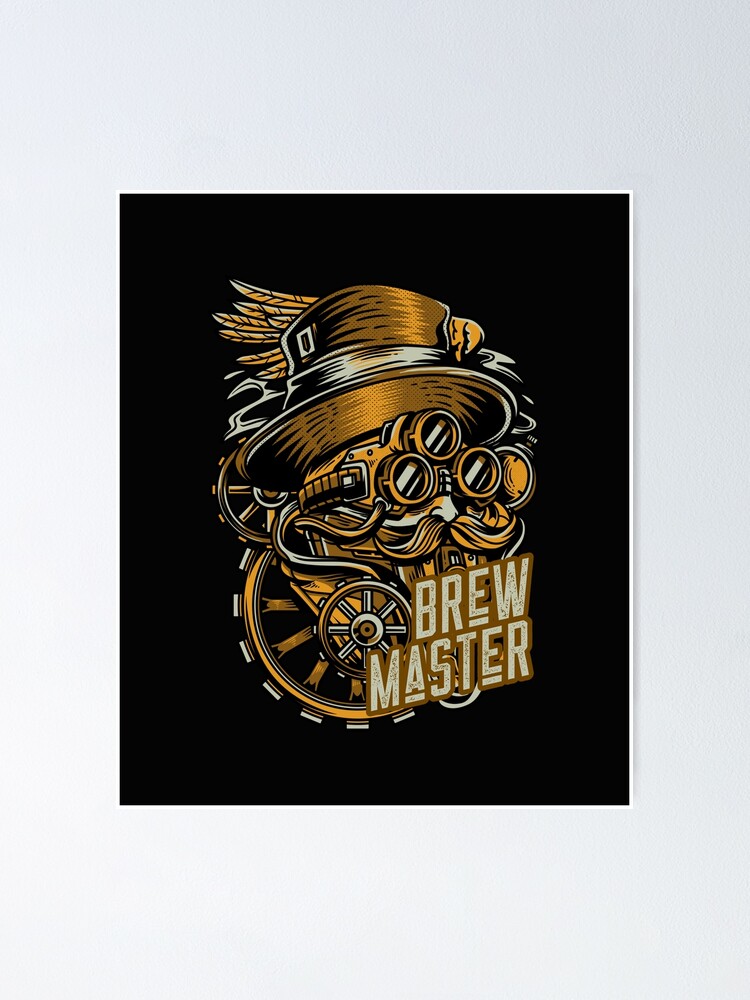The photograph showcases a steampunk-inspired piece of art centrally positioned on a white canvas backed by an eggshell white wall, with only the edges of the true white canvas visible. The artwork is dominated by a black background and features a detailed portrayal of a man's face with a distinctive steampunk aesthetic. The man wears multi-lens goggles, including an additional lens positioned between the main pair, all surrounded by a headband. A prominent, long orangey-gold mustache adorns his face, and his neck is obscured by the word "Brewmaster" in white text. He dons an old pilgrim-style top hat, complete with a buckle and feathers protruding from the back. Interwoven within the portrait are mechanical gears, with two visible behind the head and one integrated into the "Brewmaster" text. The color palette of the artwork is primarily composed of browns, yellows, tans, and golds, resembling the hues of beer, lending a vintage, sepia-toned feel to the piece. The entire composition radiates a professional quality, evoking an air of intricate craftsmanship and thematic cohesion.